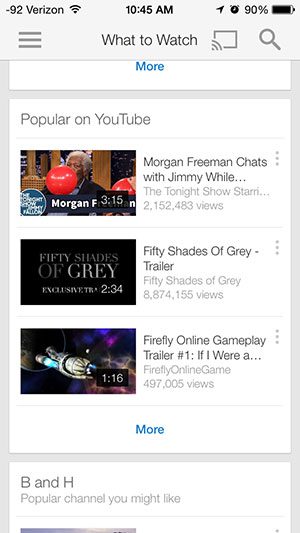The image depicts a mobile app or website interface focused on video content. At the very top, there's a heading that reads "What to Watch," followed by a section labeled "Popular on YouTube." Below this, another section appears marked "B&H, popular channel you might like," introducing more video content, though it's unclear if all videos are from YouTube. The interface then displays three specific video thumbnails:

1. **Morgan Freeman Chats with Jimmy Fallon**:
   - Thumbnail: Morgan Freeman inflating a red balloon.
   - Video Duration: 3 minutes and 15 seconds.

2. **Fifty Shades of Grey Trailer**:
   - Thumbnail: A simple black background with "Fifty Shades of Grey" in grey text.
   - Views: 8.8 million.

3. **Firefly Online Gameplay Trailer**:
   - Thumbnail: A computer-generated spaceship in space.
   - Video Duration: 1 minute and 16 seconds.

Despite the YouTube references, the app's overall functionality suggests it might aggregate video content from various sources, creating an all-in-one video viewing experience.